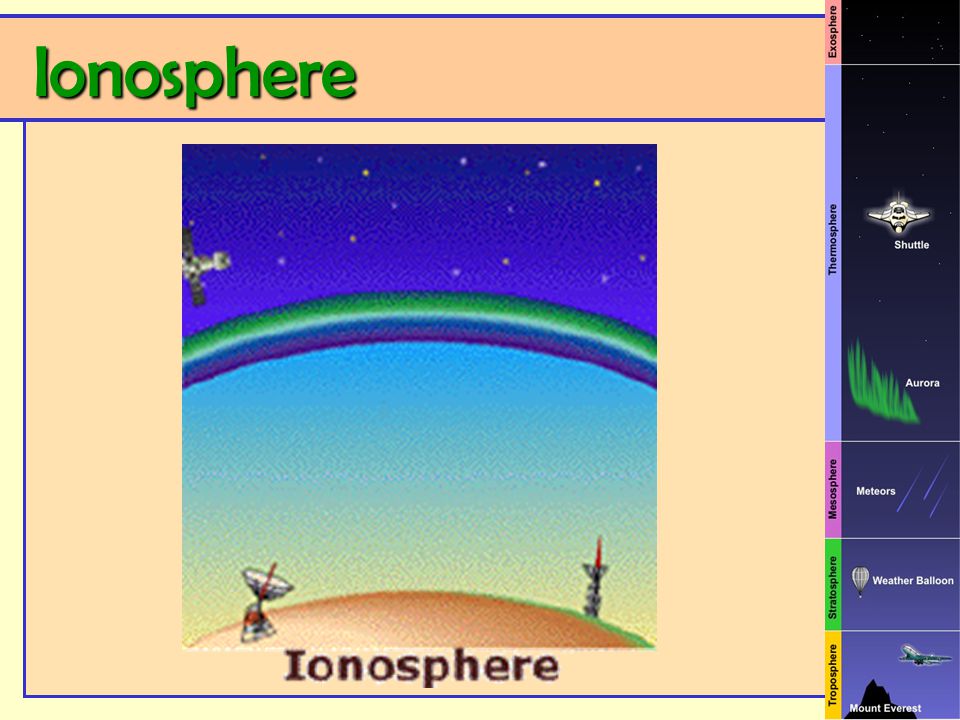The image, apparently a screenshot from a computer slide resembling a PowerPoint presentation or gaming platform, features a detailed diagram of atmospheric layers with a light pink background. A darker pink rectangle at the top hosts the title "ionosphere," written in green letters with a blue border. Centered below, the main visual includes a blue sky with stars, a plane flying left, and a green, white, and blue arc, symbolizing the ionosphere layer. Two gray instruments with red beams face upward from a sand-colored hill at the bottom of this section, described again with "ionosphere" in dark letters.

To the right, a vertical rectangle with a night-sky gradient serves as a detailed atmospheric cross-section. Near the bottom is Mount Everest labeled "troposphere," above which is a weather balloon in the "stratosphere." Higher up are bluish-purple meteors streaking through the "mesosphere," and the green aurora borealis at the bottom of the "thermosphere," where a labeled white shuttle flies. The topmost dark section denotes the "exosphere." The colors and labels, including shuttle, aurora, meteors, weather balloon, and Mount Everest, are depicted with diverse hues such as purple, yellow, tan, green, blue, black, and white, creating a vivid and comprehensive representation of Earth's atmospheric layers.